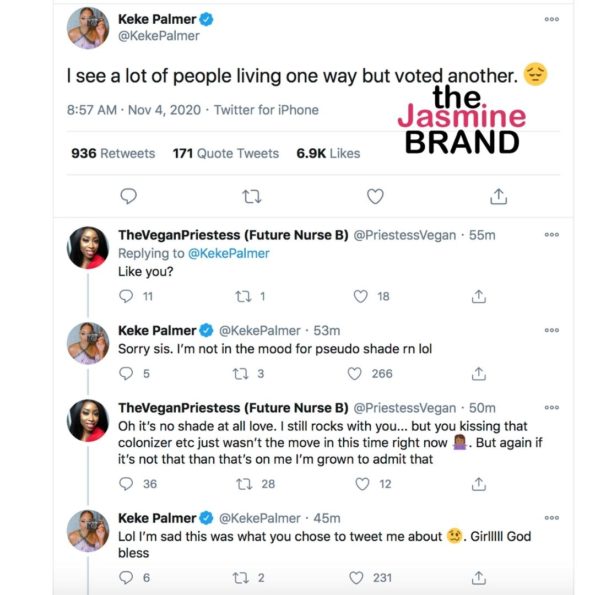This is a detailed caption for an image featuring a Twitter conversation screenshot. The image includes a watermark reading "the Jasmine brand," where "the" is in lowercase black letters, "Jasmine" is in pink letters, and "BRAND" is in all uppercase black letters.

The primary tweet is from the verified account of actress Keke Palmer (@KekePalmer), marked by a blue checkmark. The tweet, posted at 8:57 AM on November 4, 2020, via Twitter for iPhone, reads: "I see a lot of people living one way but voted another." The tweet has garnered significant engagement with 936 retweets, 171 quote tweets, and 6.9 thousand likes.

The conversation features a reply from a user named "The Vegan Priestess. Future Nurse Bee," posted 55 minutes after Keke's tweet. The reply says, "Like you," and has received 21 retweets, 18 likes, and 5 replies. In a subsequent interaction, the same user further clarifies: "Oh, it's no shade at all, love. I still rocks with you. But you kissing that colonizer etc. just wasn't the move in this time right now. But again, if it's not that, then that's on me. I'm grown to admit that." This follow-up reply has 28 retweets and 12 likes.

Keke Palmer responds with: "This is what you chose to tweet me about. 🙃 Girl, god bless," which has received 6 replies, 2 retweets, and 231 likes.